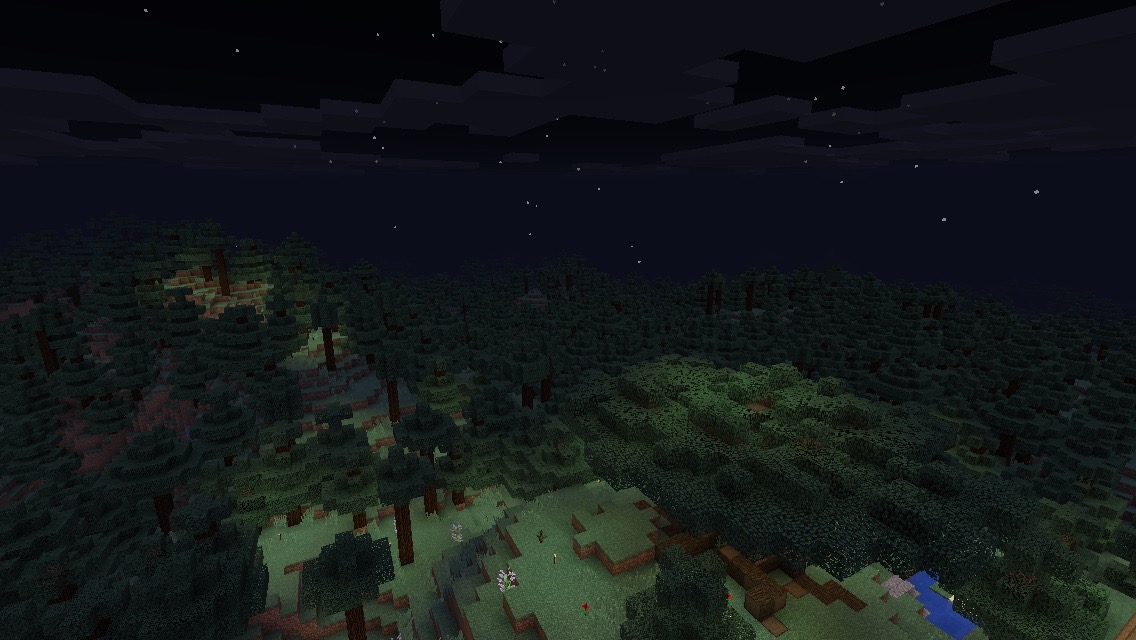The image, resembling a screenshot from a video game, portrays a blocky, pixelated landscape reminiscent of Minecraft. The rectangular frame, oriented horizontally, splits nearly in half, with a dark, starlit sky dotted with light clouds at the top. Beneath the sky stretches a green expanse of trees, bushes, and grassy terrain, extending the entire width of the image. The forest appears dense and vast, with some areas showing open patches of grass. The vegetation, mountains, and other elements exhibit a distinct blocky, puzzle-piece appearance, typical of many video games. Towards the bottom right, a small, pixelated body of water can be seen, occupying a tiny fraction of the image. In the bottom-left area, there are grayish, stone-like objects adding to the variety of the terrain. The scene lacks any buildings, emphasizing its natural, uninhabited state, with layered, stacked green landscapes creating a cartoon-like aesthetic.